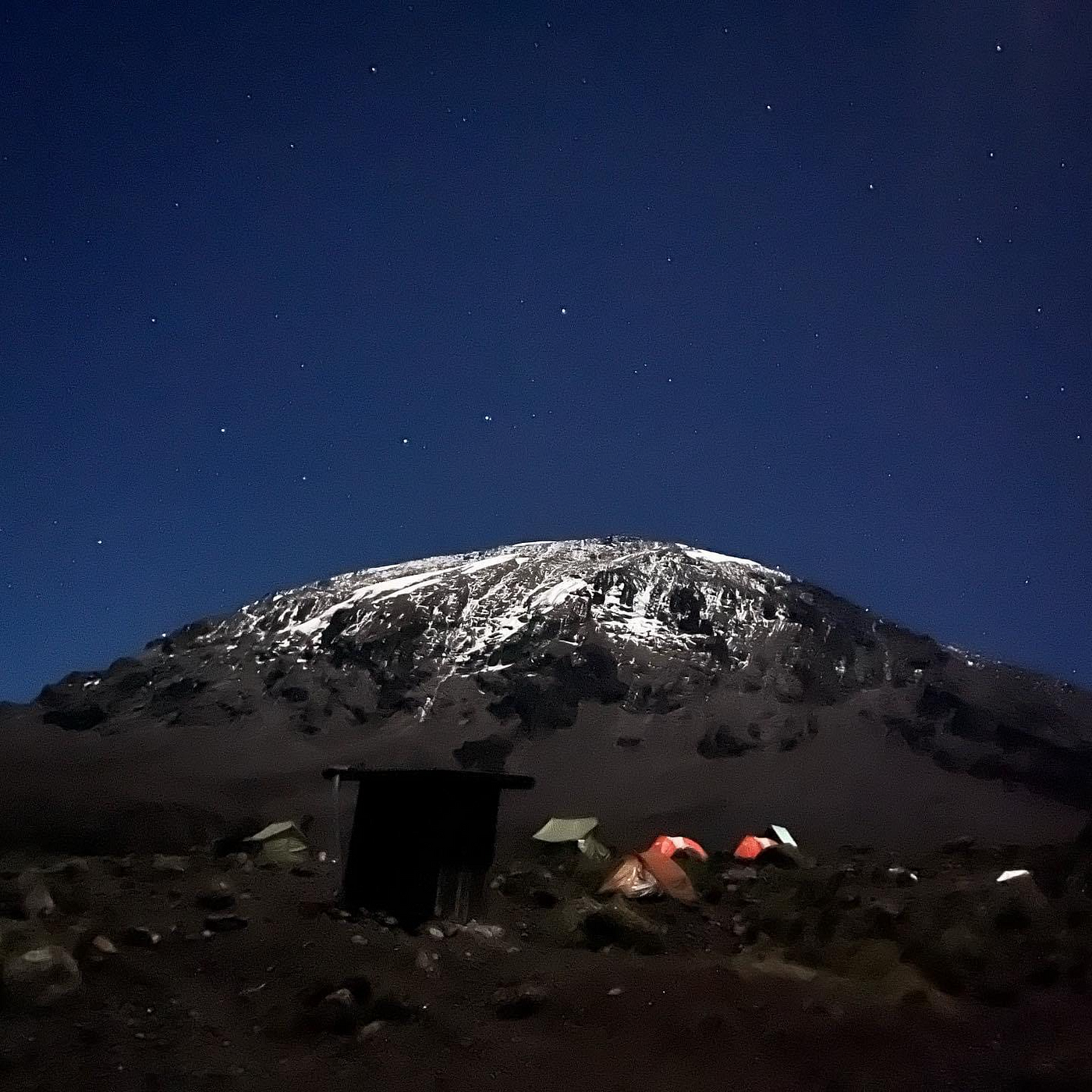In this square image, we are presented with a potentially digitally enhanced photograph of a stunning mountain scene under a dark night sky. The sky on the left side of the image is sprinkled with numerous stars, contributing a serene and ethereal ambiance to the setting. Centered in the image is a rounded mountain, dark in color, accentuated by scattered patches of bright snow near its summit. The base of the mountain transitions into a relatively flat expanse of ground that hosts a small, illuminated campground. The campground features four tents on the right side: three of which are red and one green. An additional green tent is pitched on the left side of the image. Dominating the center of the campsite is a rectangular brown structure, likely an outhouse, though its exact purpose is indistinguishable due to the low light of the nighttime photograph. The scene is a harmonious blend of natural beauty and human presence, captured under the vast expanse of a star-studded sky.